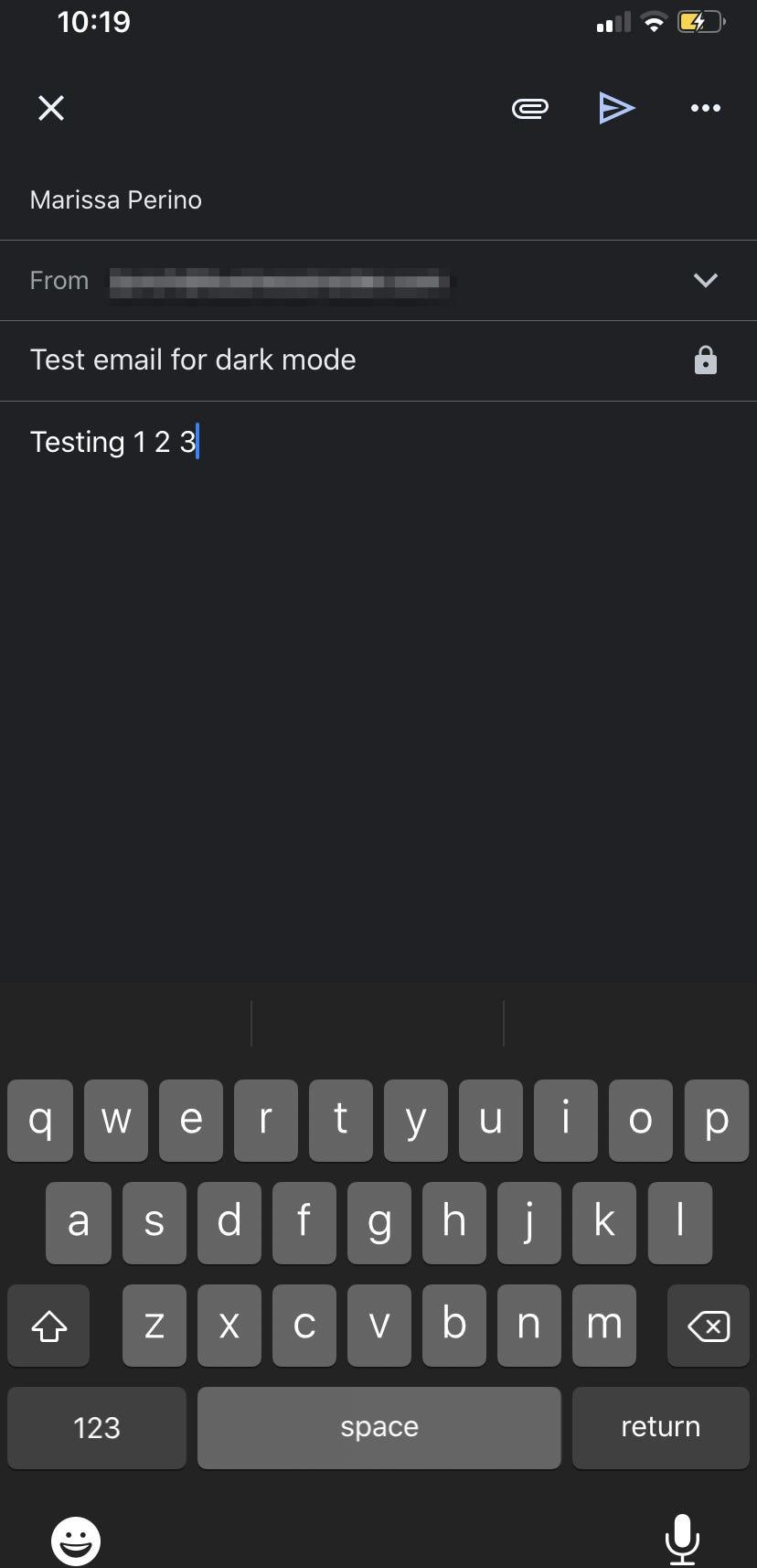The image depicts a black smartphone screen set against a black background. In the upper right corner, a partially filled yellow battery icon indicates about 50% charge. The device shows a moderate signal strength, and the time displayed is 10:19. Below the time, an X mark is visible. 

Adjacent to the X, several icons are noticeable: one is an inward curving oval shape, another is a blue right-facing arrow resembling a triangle with an inner detail, and there are three horizontal bars lined up vertically. 

At the top of the screen, the name "Marissa Perino" is displayed, followed by the word "from" with the sender's information grayed out and a dropdown arrow on the right. The subject line reads "test email for dark mode," accompanied by a lock icon. The body of the email begins with "testing one, two, three," and a blue bar appears right next to the number three.

At the bottom of the screen, the virtual keyboard is visible, showing text being typed. Below the keyboard's number key (1, 2, 3) is a white smiley face icon, and under the return key is a white microphone icon.